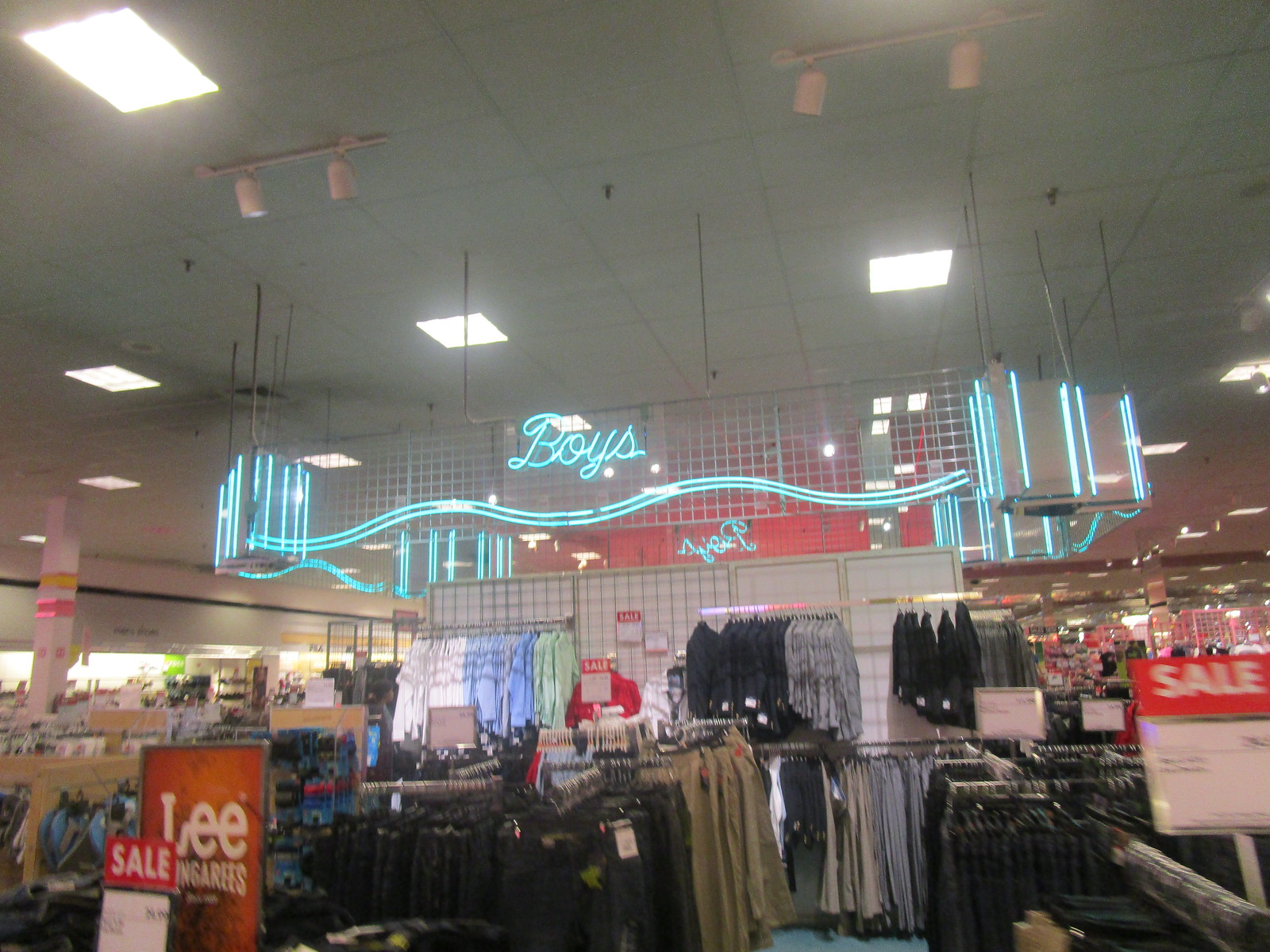The image depicts the boys' section of a large, possibly less expensive department store, characterized by its high ceilings and utilitarian lighting fixtures. A prominent neon blue sign, outlined in white and turquoise, clearly marks the boys' section. Sale signs, with white text on red backgrounds, are eye-catching and scattered throughout the area. Various clothing items, including shirts and pants, are organized on racks at different heights and on T-bar stands. In the background, there is a vintage-looking "Lee Dungarees" sign, indicative of an older image given the rare use of the term "dungarees" today. The store layout includes aisles and additional sections on both sides, contributing to the open and expansive atmosphere of the department store.